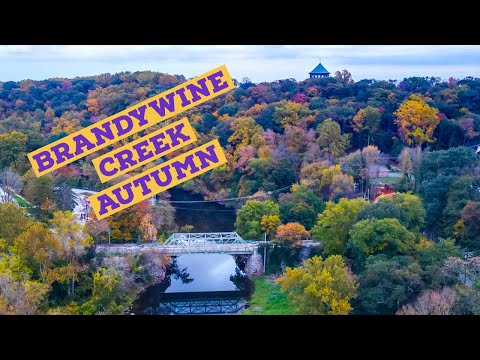This is an overhead photograph capturing the stunning autumn scenery of Brandywine Creek. The image showcases a rich, multicolored forest with trees in various shades of green, yellow, gold, red, and even purplish tones, emblematic of the fall season. Dominating the center of the image, a white steel truss bridge extends across a calm river, its reflection clearly visible in the tranquil water below. Over the scene, purple text on orange banners diagonally spells out "Brandywine Creek Autumn" in large, bold letters. Towards the background, a triangular-roofed structure peeks out above the treetops, under a beautiful clear sky. Power lines hover above the bridge, adding to the intricate details of this picturesque landscape.